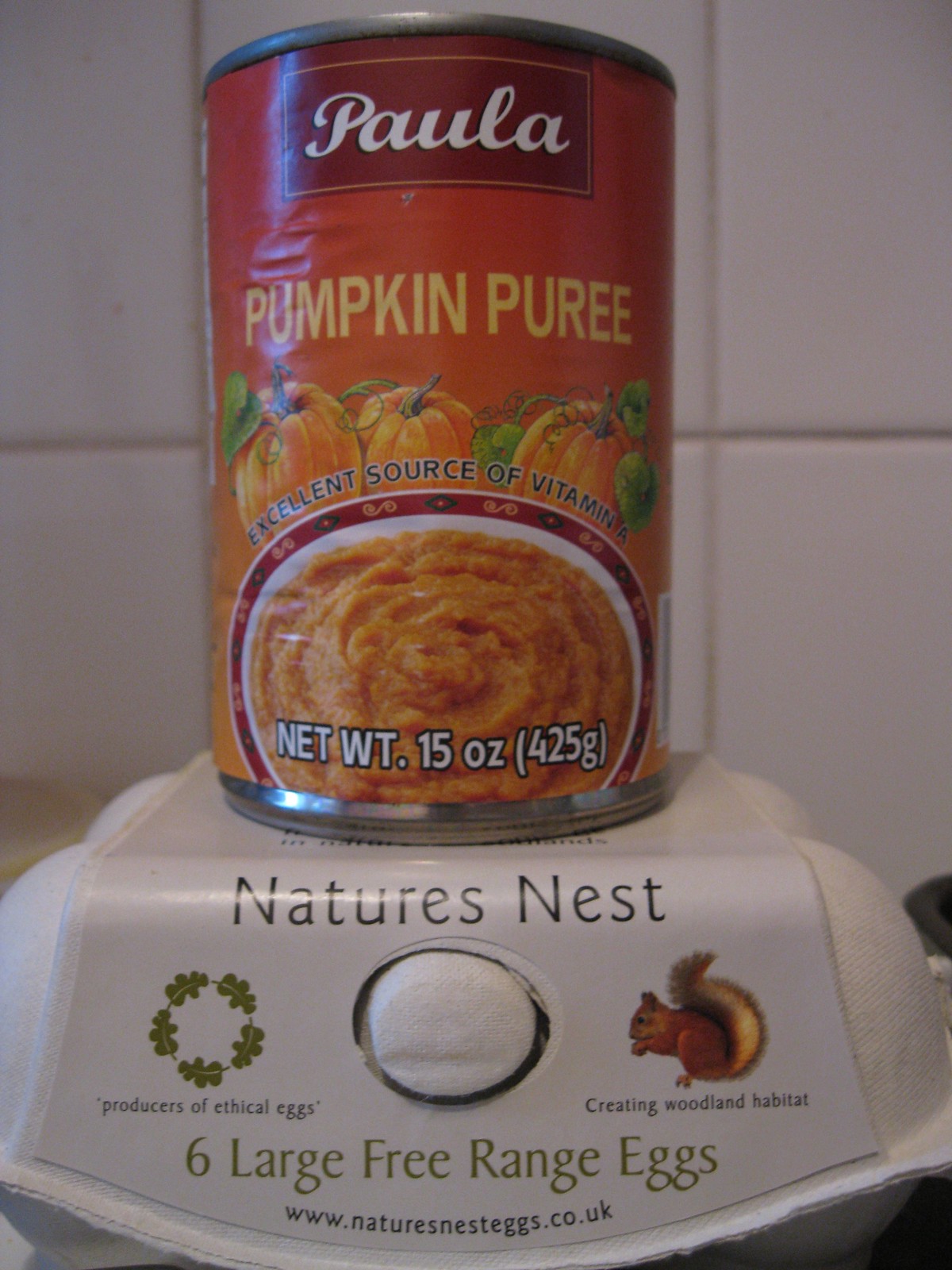A detailed and descriptive caption for the image could be:

"The image features two food products stacked together. On the bottom is a small, eco-friendly cardboard carton labeled 'Nature's Nest' containing six large free-range eggs. This carton emphasizes sustainable packaging. Positioned on top is a can of 'Paula Pumpkin Puree,' which boasts being an excellent source of Vitamin A. The can has a predominantly orange design and lists a net weight of 15 ounces (425 grams). It is unclear if the items are intended to be used together or if they were simply placed together for the photograph."